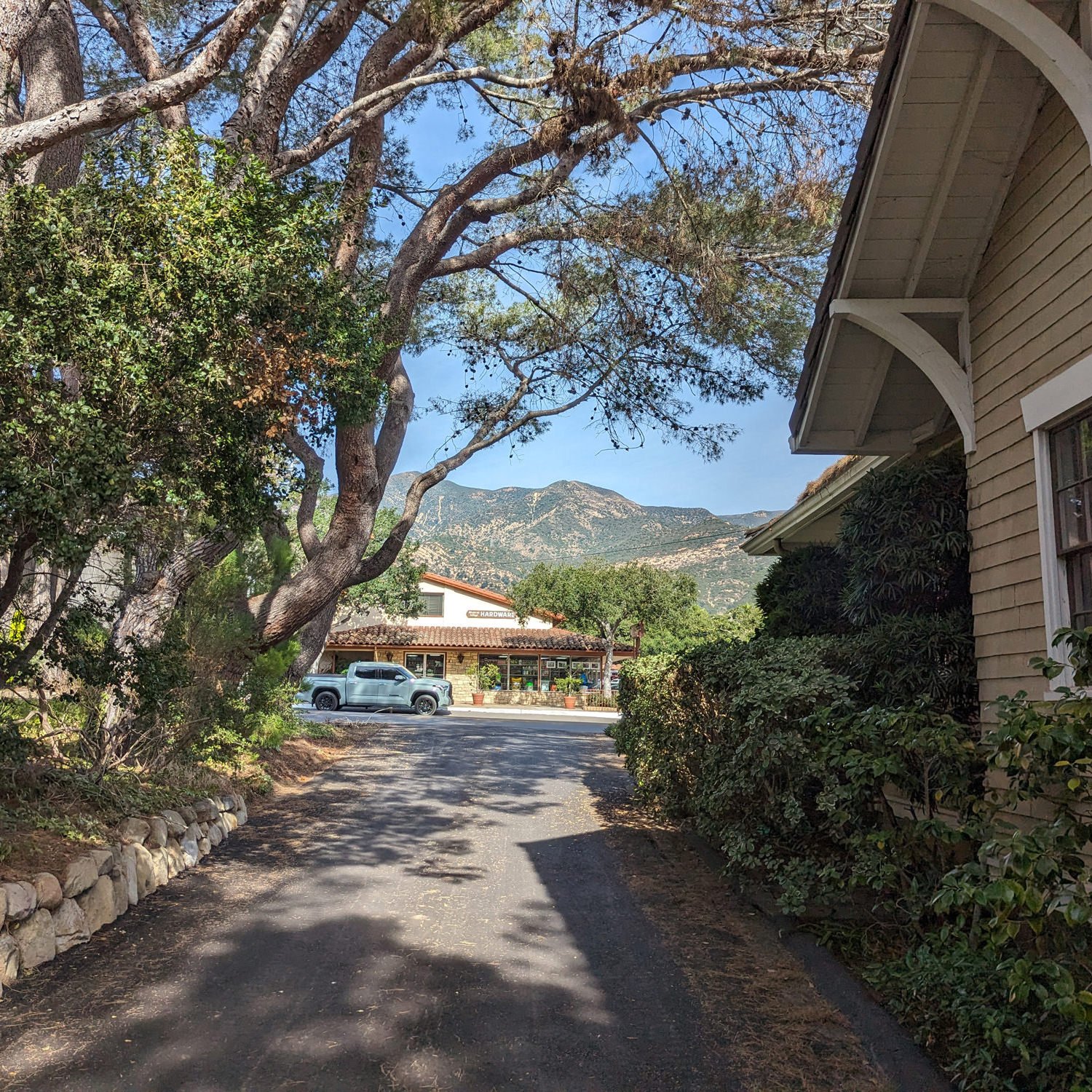The image depicts a serene, sunny day in a rural, possibly South American, mountainous region, capturing a driveway shaded by numerous trees and bordered by a stone retaining wall with well-kept grass. On the right, partially visible, is a light tan house with a window, some hedges, and a bit of its roof. The driveway leads to a street that feels more like a quiet village road than a busy urban thoroughfare. At the bottom of the driveway, across the street, stands another house with a white (or light blue) pickup truck parked in front. The background reveals an open sky and a beautiful mountain range, adding to the peaceful rural atmosphere. The vegetation, trees, and shadows cast by the bright sunlight create a picturesque and inviting scene.